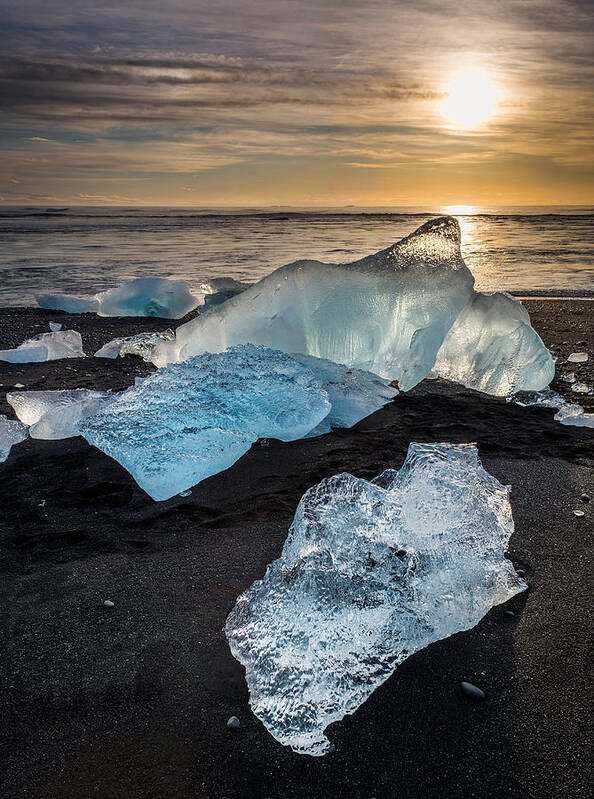The image captures a serene beach scene at sunset, with several large chunks of ice scattered across black sand, creating a striking contrast. The sizable ice formations, ranging in color from light refreshing turquoise to teal, appear translucent and clear, with some pieces jutting upward dramatically. The scene is illuminated by a bright yellow sun positioned in the top right corner of the sky, casting a soft yellow glow and enhancing the elegant, picturesque quality of the setting. The sky itself is a beautiful gradient of orange mixed with hints of blue, adorned with thin, wispy clouds. The calm, wave-free ocean gently laps the shoreline, reflecting the melting effect of the warm sun, which seems to be descending towards the horizon.